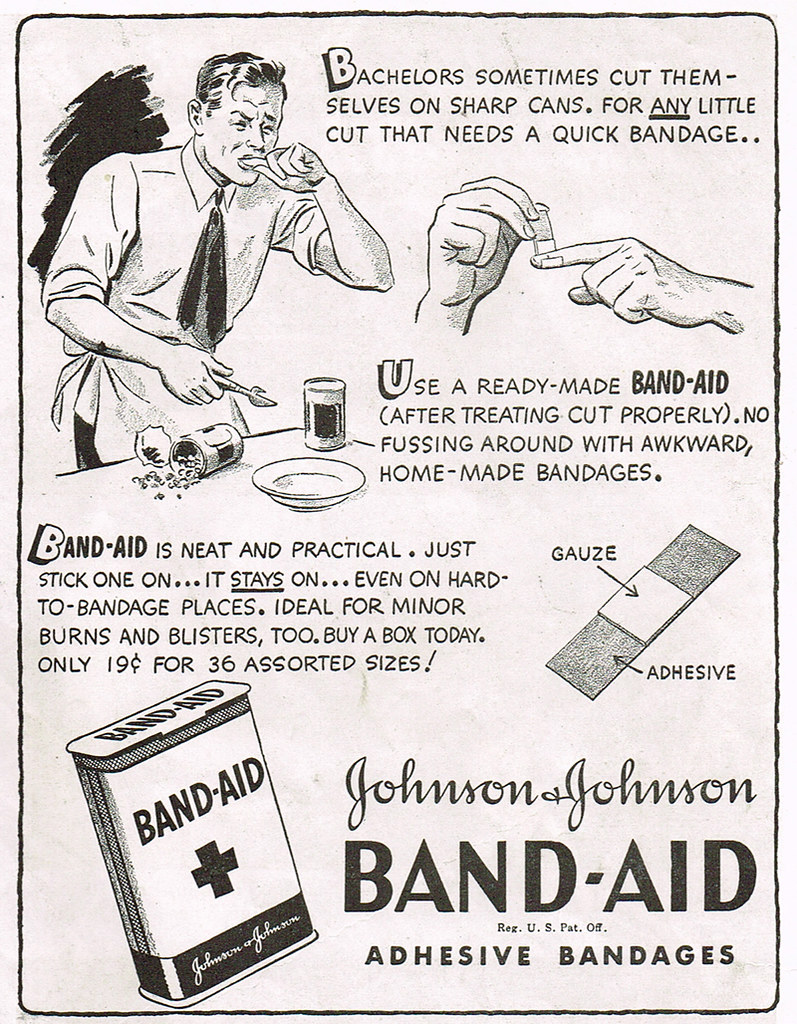This vintage advertisement, likely from the 1930s or 1940s, for Johnson & Johnson Band-Aid Adhesive Bandages, exudes the charm of a classic comic book. Illustrated in black and white, the ad features a cartoon character—a bachelor in a white shirt and tie—who has accidentally cut his finger while opening a can of vegetables. Above him, a caption reads, "Bachelors sometimes cut themselves on sharp cans. For any little cut that needs a quick bandage."

To the left of the man, a metal band-aid canister is depicted with the Johnson & Johnson logo. A detailed sequence shows the man wrapping a band-aid around his injured finger, accompanied by reassuring text: "Use a ready-made band-aid after treating the cut properly. No fussing around with awkward homemade bandages." An illustration of a band-aid follows, highlighting its practical and neat design, along with the adhesive properties.

Further text assures the reader, "Band-Aid is neat and practical. Just stick one on—it stays on even on hard-to-bandage places. Ideal for minor burns and blisters too." Concluding the advertisement, it encourages viewers to "Buy a box today for only 19 cents for 36 assorted sizes," underscoring the affordability and convenience of the product. The ad also proudly notes the product's registered status with the U.S. Patent Office.